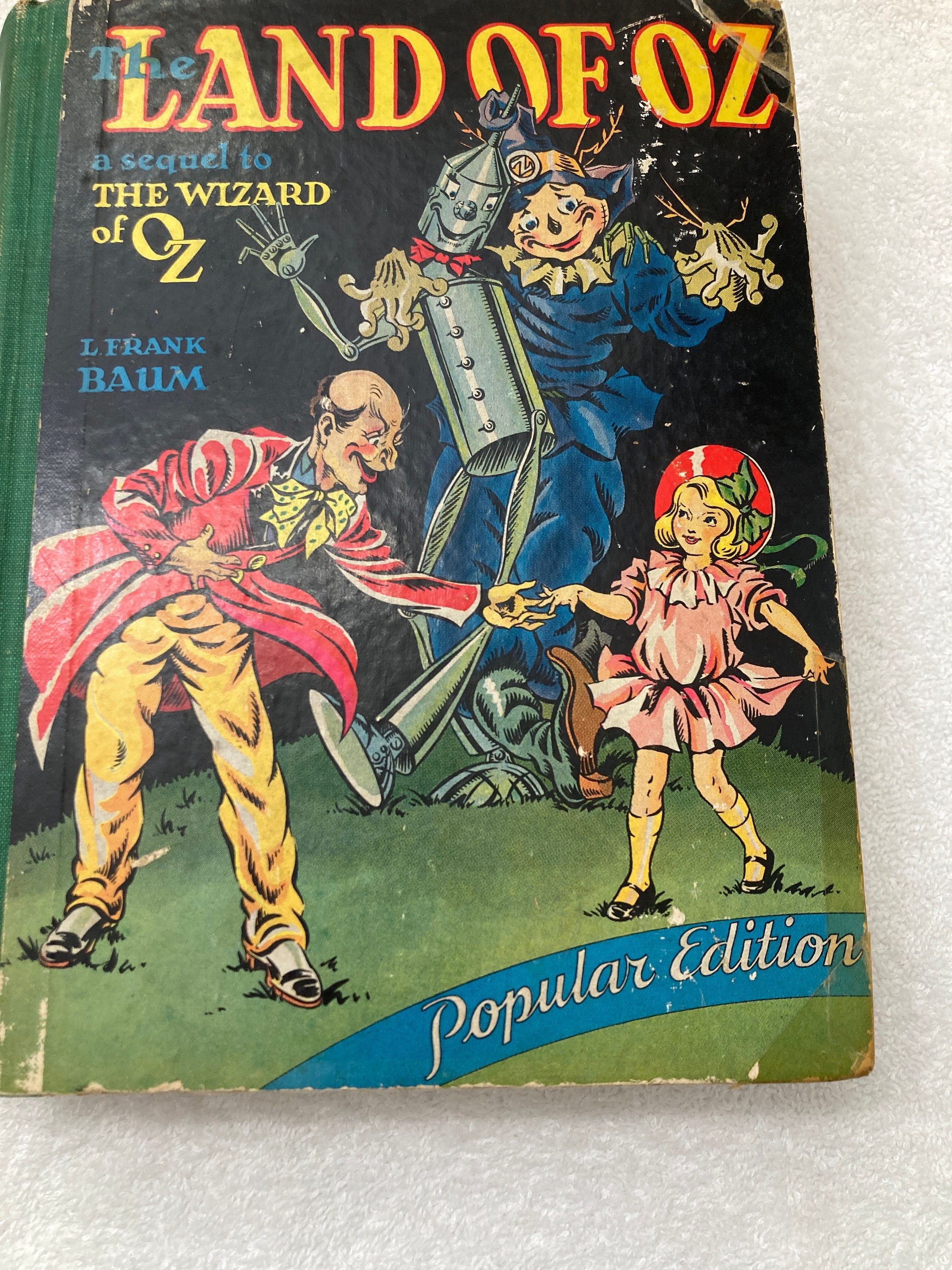The photograph is a portrait-style image of a vintage children's book titled "The Land of Oz: A Sequel to The Wizard of Oz" by L. Frank Baum. The book's well-worn cover, marked with numerous scuffs and signs of age, speaks to its longtime usage. This edition is notably labeled as a "Popular Edition" in script at the bottom of the cover. The vibrant illustration features Dorothy, depicted with short blonde hair adorned with a green bow and red hat, wearing a pink dress paired with yellow knee socks and black Mary Jane shoes. She is shown shaking hands with a character in a red suit jacket and yellow pants, presumably Mr. Oz, who has a somewhat nefarious expression. Surrounding them are the Scarecrow, dressed in a blue outfit, and the Tin Man, sporting a red bow tie, both walking arm-in-arm. The overall scene is cheerful, yet with an unmistakable vintage charm that predates the more familiar movie adaptations.